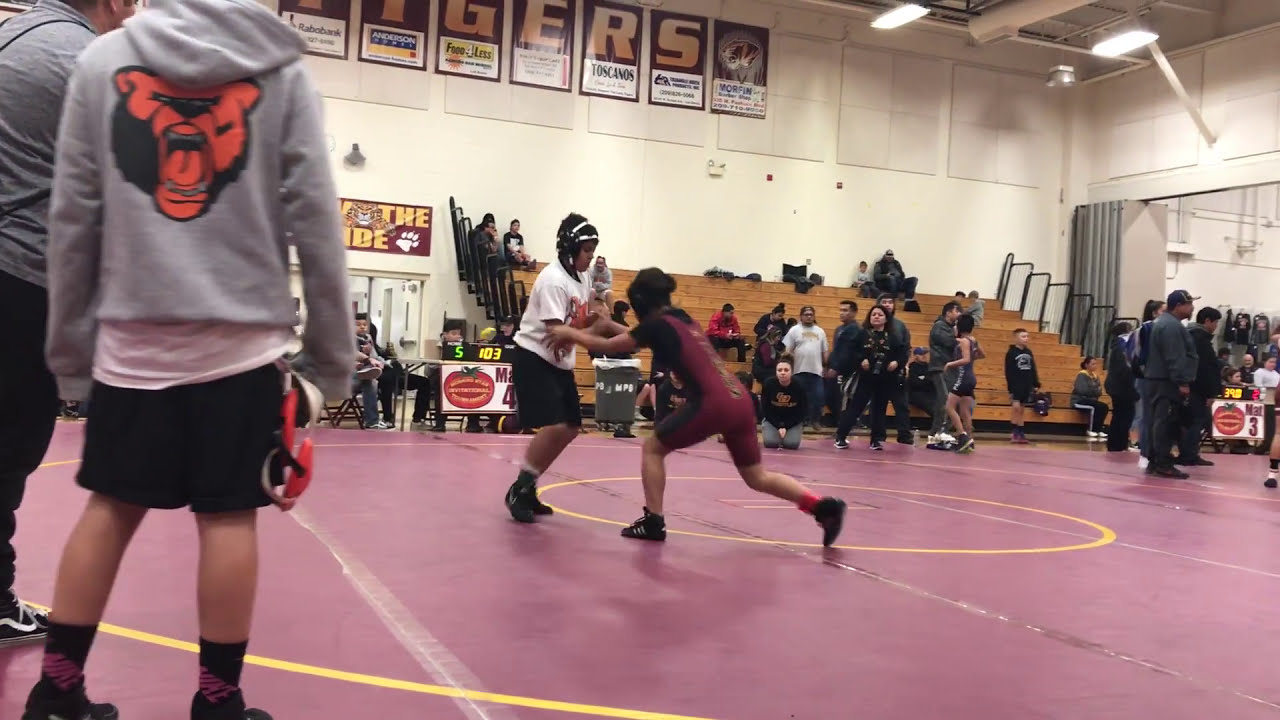In a bustling gymnasium with crimson flooring and yellow stripes, two wrestlers command the center of the scene, locked in a fierce grapple near a yellow circle on the floor. The wrestler on the left, clad in a white t-shirt, black shorts, and white and black headgear, defends against a lunge from their opponent, who wears a striking black and red leotard and black Adidas shoes. Flanking the wrestling match, two spectators stand closely together—the one on the left sports a gray hoodie adorned with a red and black bear on the back, a white t-shirt underneath, black shorts, black socks, and black shoes, while their companion dons a gray shirt, black pants, and black and white sneakers.

Surrounding the match, a lively crowd fills the brown bleachers accentuated with black railings, while others are seated at tables marked with numbers, perhaps judges diligently watching the match. The walls of the gym are white, adorned with banners proudly displaying the word "TIGERS" in bold orange letters on black backgrounds, alongside a larger sign featuring "THE PRIDE" with an image of a tiger. The diverse audience, dressed predominantly in dark clothing and some in hats, adds a sense of anticipation and excitement to the energetic atmosphere.